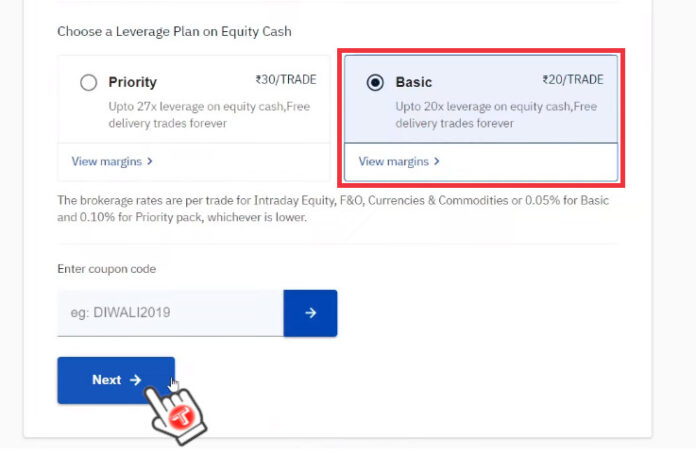In this emergency context, consider opting for a leverage plan with equity cash priority. This plan offers 27 times leverage on equity cash trades at a rate of 30 rupees per trade, along with free delivery trades forever. Alternatively, the basic plan provides up to 20 times leverage on equity cash while maintaining the same benefit of free delivery trades. Brokerage rates are charged per trade for intraday equities, futures & options, currencies, and commodities or calculated at 0.05% for the basic plan and 0.1% for the priority pack, whichever amount is lower. At the bottom of the screen, there is an option to enter a coupon code (e.g., 'diwali2019'), accompanied by a hand cursor icon hovering over the "Next" button.